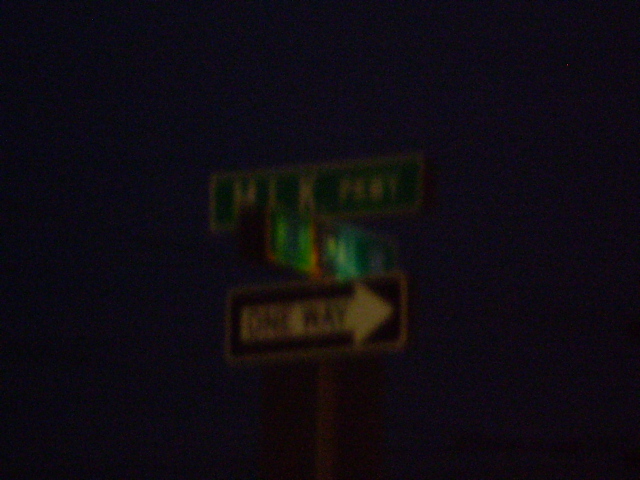In this slightly blurry image, we observe an intersection viewed from below. At the very bottom, the backside of a square black sign is partially visible. Mounting this sign is a brown pole, which also supports a rectangular sign above it. This sign reads "One Way" with a white arrow pointing to the right. Above it, a green road sign displays "I'm OK," and directly below it, another green sign points in the opposite direction. The background of the image is dominated by a deep, almost midnight blue sky, stretching from edge to edge.